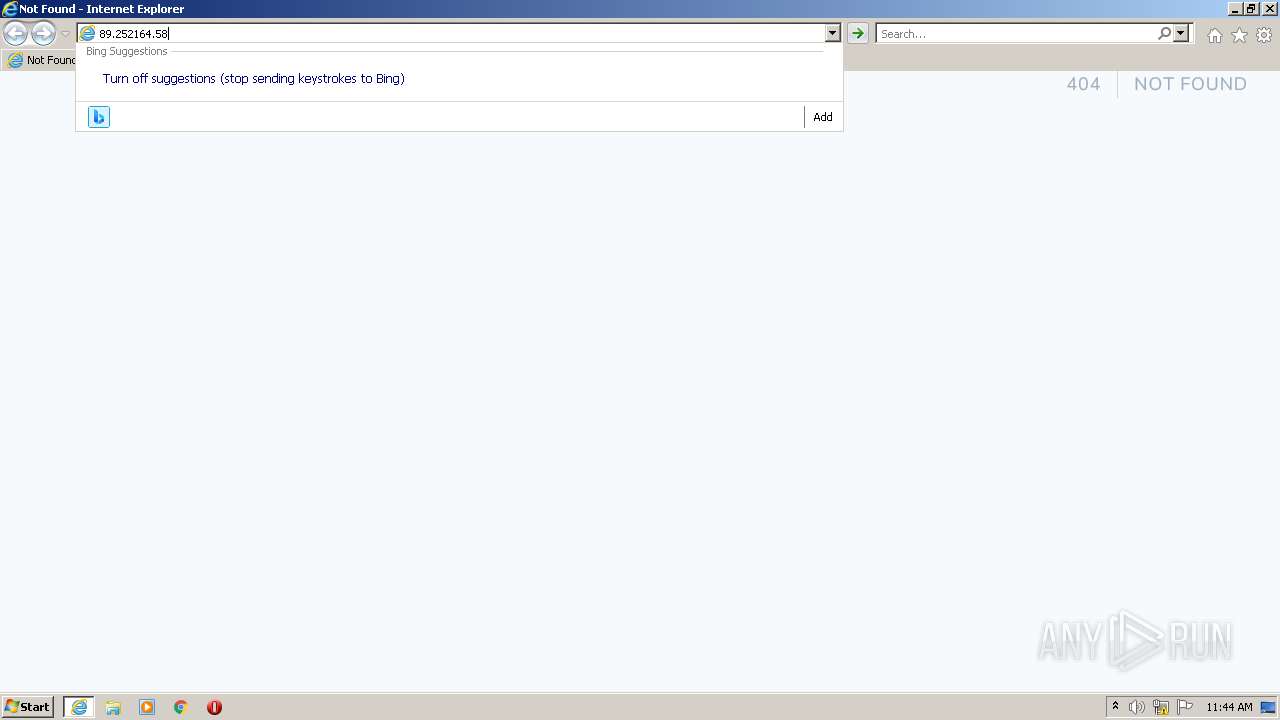### Detailed Image Caption:

This image appears to be a screenshot taken from an older version of Internet Explorer. The top of the screenshot features a slender blue bar, which displays the Internet Explorer logo alongside the text "Not Found - Internet Explorer" in white. 

In the upper right corner of this blue bar, there are three distinct icons: 
1. A black bar with a dash at the bottom, representing the minimize function.
2. An icon depicting one box overlapping another, signifying the resize function.
3. A gray box with a white 'X', used for closing the window.

Below this blue bar, there is a gray toolbar housing various navigation and function elements. It includes backward and forward arrows for navigation, and an IP address, "89.252.164.58," displayed in black text. This is followed by a search box, which contains the word "Search". Adjacent to this box are several icons: a home icon, a store icon, and a gear icon.

Beneath the search box, there is blue text that reads "Turn off suggestions, stop sending keystrokes to Bing."

The main portion of the screen displays a blank white page. In the upper left corner of this blank page, ther is "404 - NOT FOUND" in all uppercase gray text, indicating that the requested page could not be found. The lower right corner of the page contains the text "ANY.RUN."

At the bottom of the screenshot, there's another gray bar—the Windows taskbar. On the left side, you can see the Windows Start button, followed by several icons: 
1. Internet Explorer
2. A file folder
3. A VLC media player icon
4. Another Windows icon
5. A red circle with a '1' in its center, likely indicating a notification.

In the lower right corner of this taskbar, several system icons are visible, including those for audio settings, battery status, a white flag (potentially indicating the Action Center), and the time, which is shown as "11:44 AM."